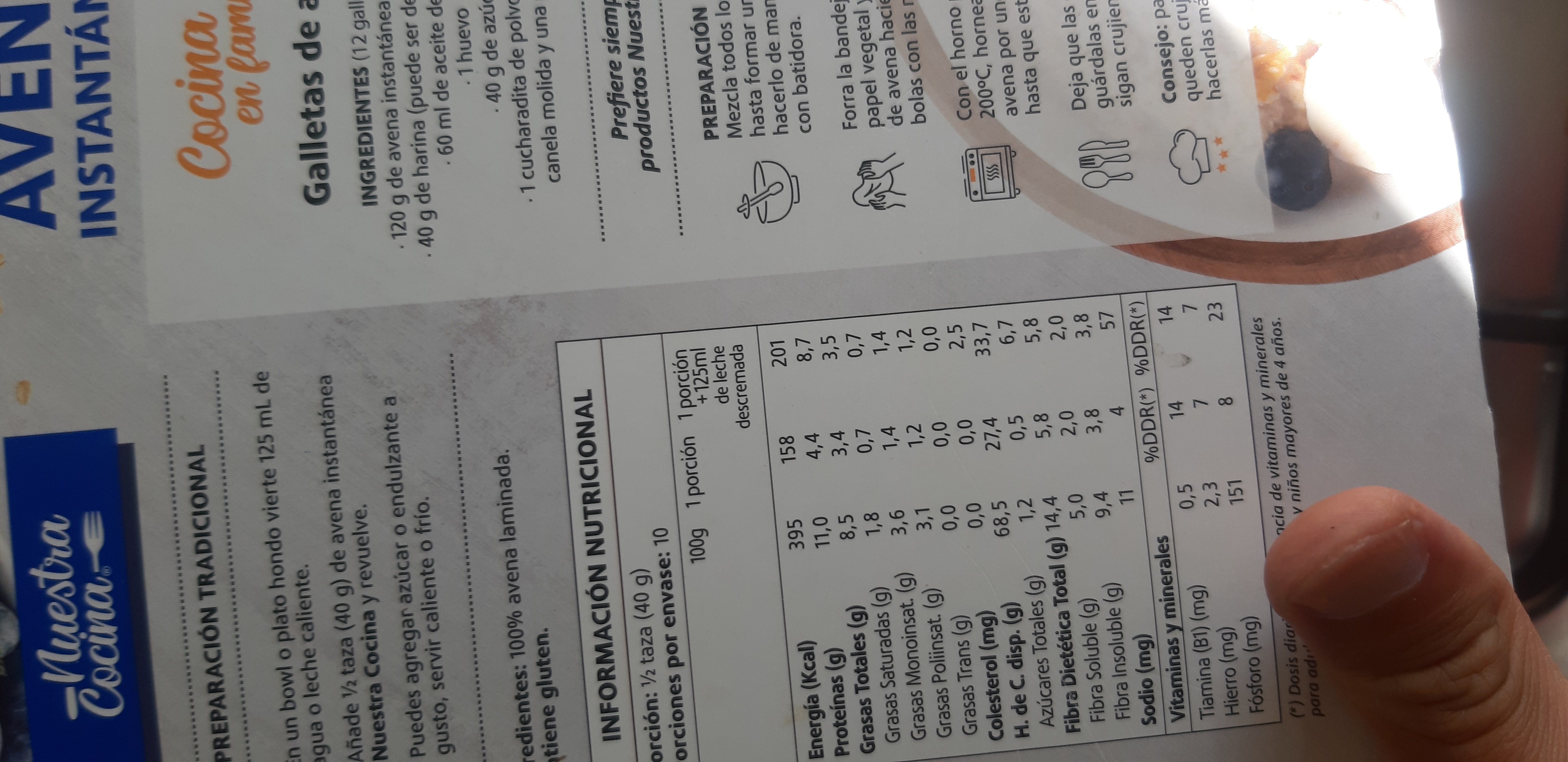A detailed caption for the image:

"The image shows a horizontal menu lying on its side, with a large thumb visible in the bottom right-hand corner, as if the person were holding it upright. The menu is written in Spanish and appears to focus on food, featuring a significant section dedicated to nutritional information. The predominant font color is black on a white background, with a contrasting blue title at the top that reads 'Nuestra Cocina.' Some text on the right is partially obscured and unreadable. The menu possibly pertains to a ready meal, given the inclusion of a 'preparation' section, suggesting it can be purchased and heated in a microwave."